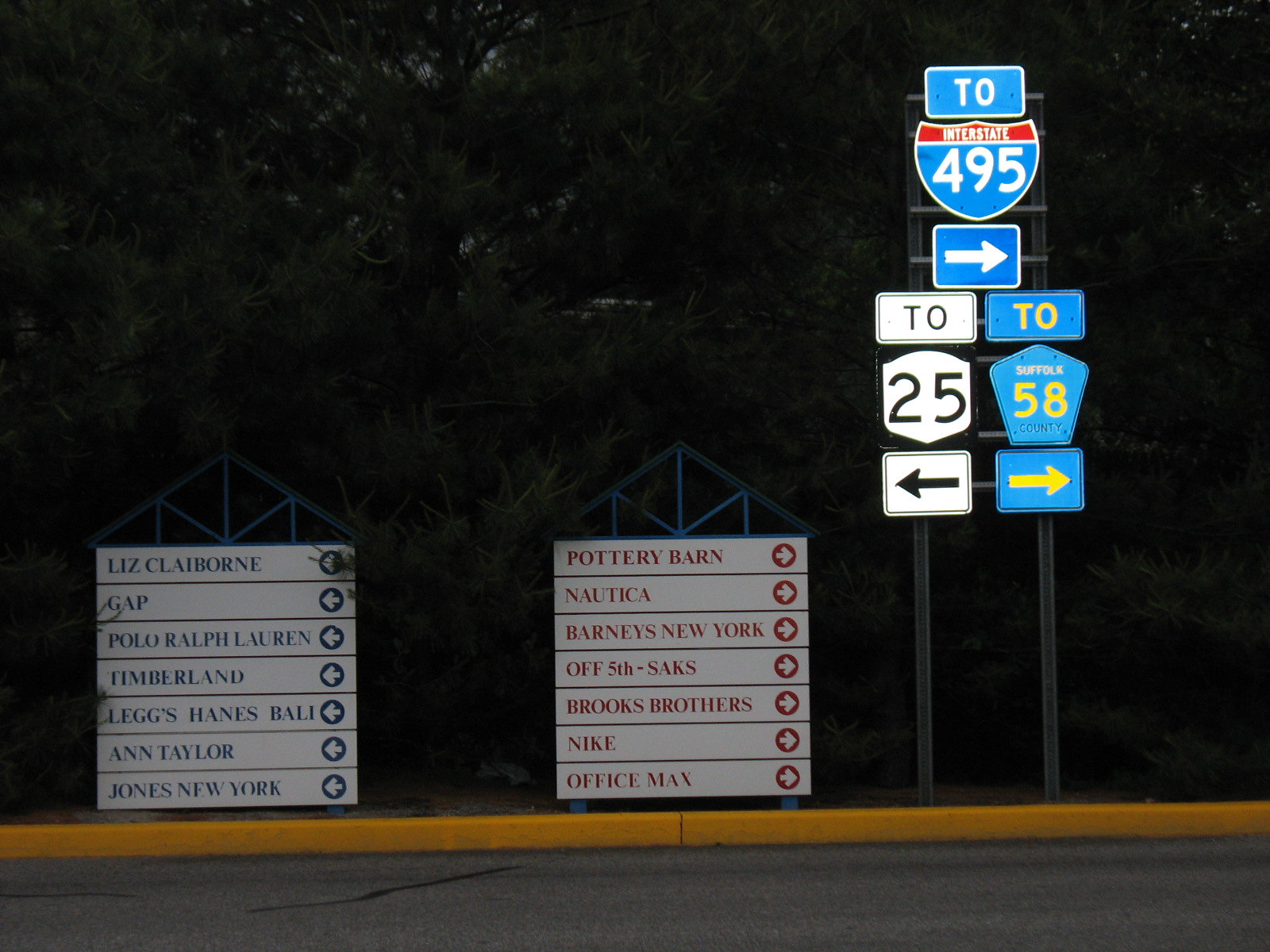This photo captures a collection of directional signs within a shopping mall complex. On the right side of the image, a large street sign directs motorists to Interstate 495 and Suffolk Route 58, both indicating a rightward direction with corresponding arrows. Adjacent to this street sign is another directing travelers to Route 25, with an arrow pointing to the left.

The photo also features several directional signs for stores. Shops indicated to the right include Pottery Barn, Nautica, Barney's New York, Saks Off 5th, Brooks Brothers, Nike, and OfficeMax. Stores located to the left include Liz Claiborne, Gap, Polo Ralph Lauren, L'eggs, Hanes Bali, Ann Taylor, and Jones New York. The comprehensive signage reflects the mall's organization, helping visitors navigate to their desired destinations efficiently.